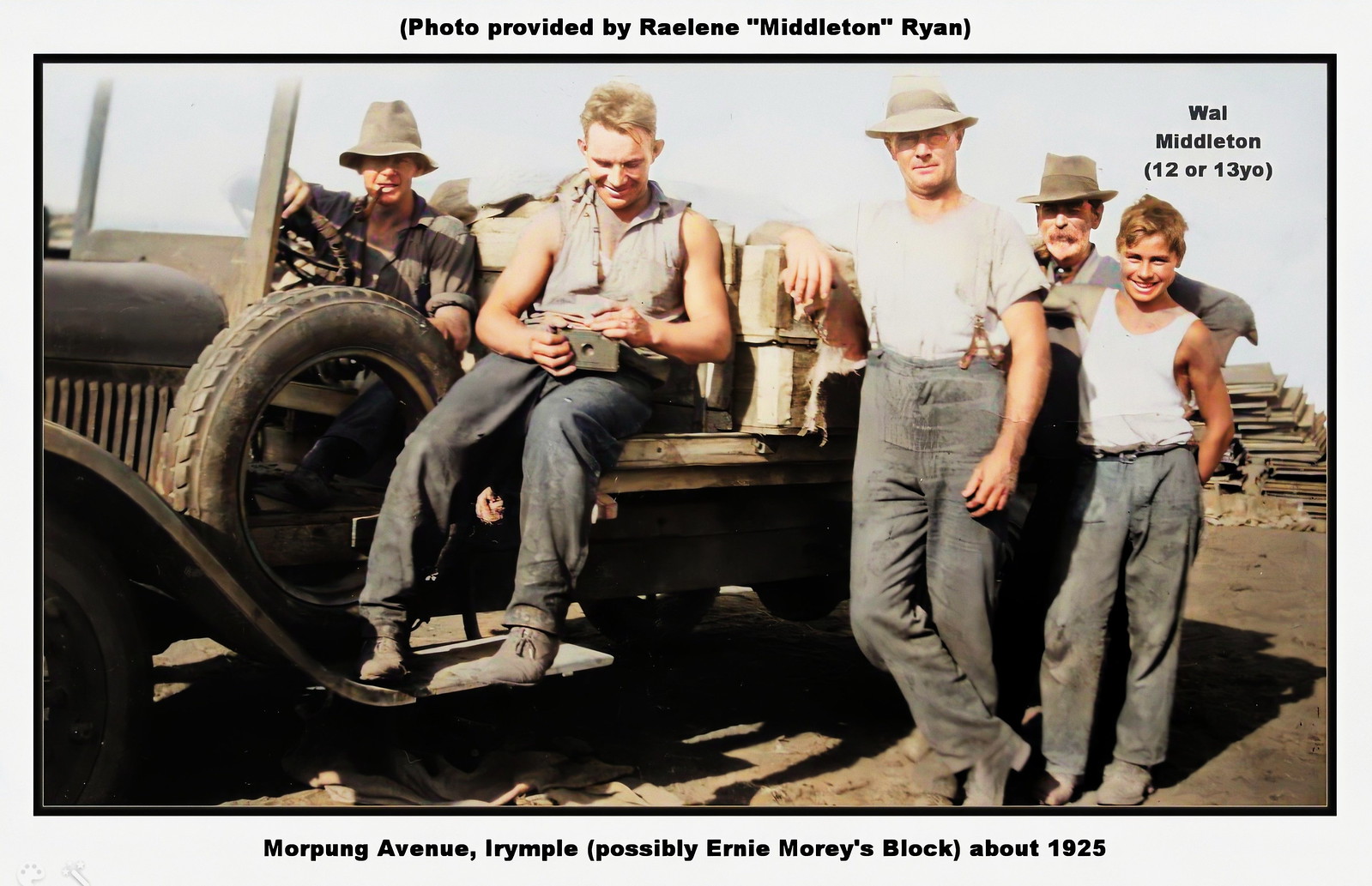This photograph, provided by Raylene Middleton Ryan and dated around 1925, captures a rustic scene on Moorpong Avenue, Earrimple, possibly at Ernie Morey's block. Despite being an image from 1925, the photograph appears in color, suggesting it may have been colorized or touched up. The scene presents five individuals embodying a rugged, perhaps hardworking ethos, underscored by their dirty, worn-out clothing consisting of old pants and t-shirts. 

Three of the men wear hats, and two sit inside an old, topless jeep, evoking curiosity about the activities they might be engaged in. One of these men, possibly an older individual sporting a Yosemite Sam mustache and a hat, seems to be fixated on something in a box, perhaps reading letters, with something resembling a pipe hanging from his mouth. Another man in the jeep, distinguished by his cut-off collared shirt unbuttoned most of the way, also appears absorbed in this activity.

Standing next to the jeep are the remaining three individuals, among whom is a young boy, identified as Whale Middleton, around 12 or 13 years old, clad in a white tank top and jeans, looking scruffy like the others. The other men, described in beat-up clothing, including one in suspenders and a white shirt, contribute to the atmosphere of the photograph. The surroundings hint at a warm, clear day, with no clouds visible in the sky, capturing a moment of seemingly mundane yet telling interaction among these rustic figures.